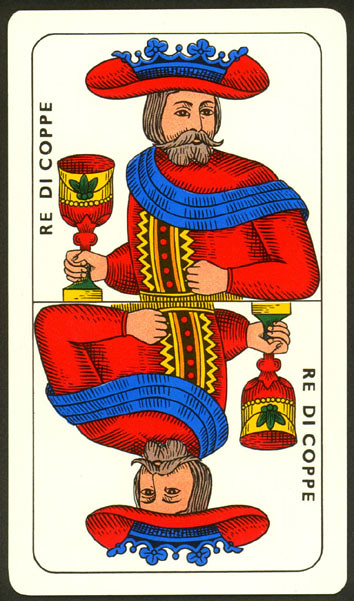This image depicts a playing card featuring an intricate and artistic illustration of a man of European descent, dressed in a distinctive red outfit. The man sports a blue shawl collar that elegantly drapes over his shoulders and back. His attire features a striking pattern of brown, red, yellow, and orange colors that cascade down the front of his clothes, reminiscent of a buttoned-up garment. He has a distinguished appearance with a mustache and gray hair, topped with a hat that matches his red and blue attire. The hat is reminiscent of a sombrero, but with a unique blue crown-like center. In his hand, he holds an ornate goblet colored in red and yellow, adorned with the depiction of a green plant. Along the right side of the image, the word "R.E.D.I.C.O.P.P.E." is inscribed, heading upwards. The entire scene is mirrored at the bottom of the card, creating a symmetrical reflection of the figure and his elaborate design.